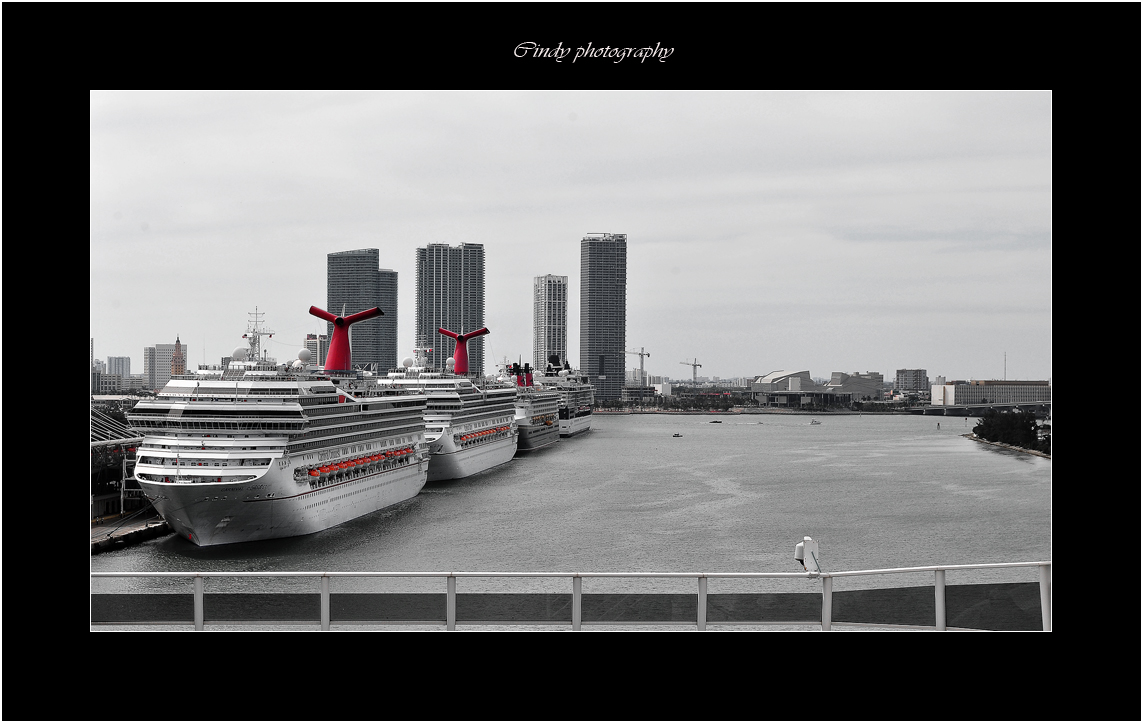The image is a professional color photograph by Gimbe Photography, framed with a black beveled mat and featuring italic calligraphy text at the top center. The scene captures a cloudy, overcast day at a bustling coastal city port. Along the left side of the image, three or four large cruise ships, adorned in silver or gray with black and red details, are docked sideways at the pier. These ships are stationary, sitting atop the blueish water, and leaving gentle watermarks behind them. In the background, the cityscape is filled with tall skyscrapers and a variety of low-rise buildings, among which construction cranes and wind turbines are visible. A white metal fence with a gray strip runs along the bottom edge of the photograph, near which a white bird perches. The overall atmosphere is serene, with no pedestrians in sight.